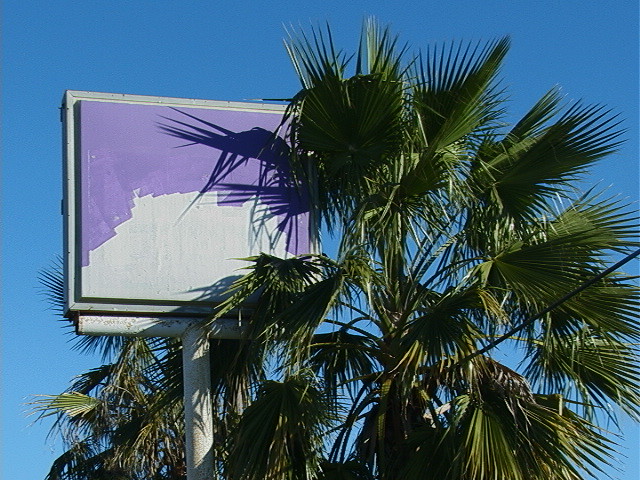In this vibrant outdoor scene, a towering palm tree stands proudly on the right, its abundant fronds displaying a rich spectrum of green hues, from deep emerald to light lime. Contrasting with the greenery, a white signpost on the left supports a square sign, partially painted in purple with a rough, unfinished texture, leaving the bottom portion starkly white. Above, the clear, brilliant blue sky forms a perfect backdrop, while a black electrical wire stretches horizontally across the image, intersecting both the sign and the palm tree, adding a touch of urban clutter to this otherwise serene setting.